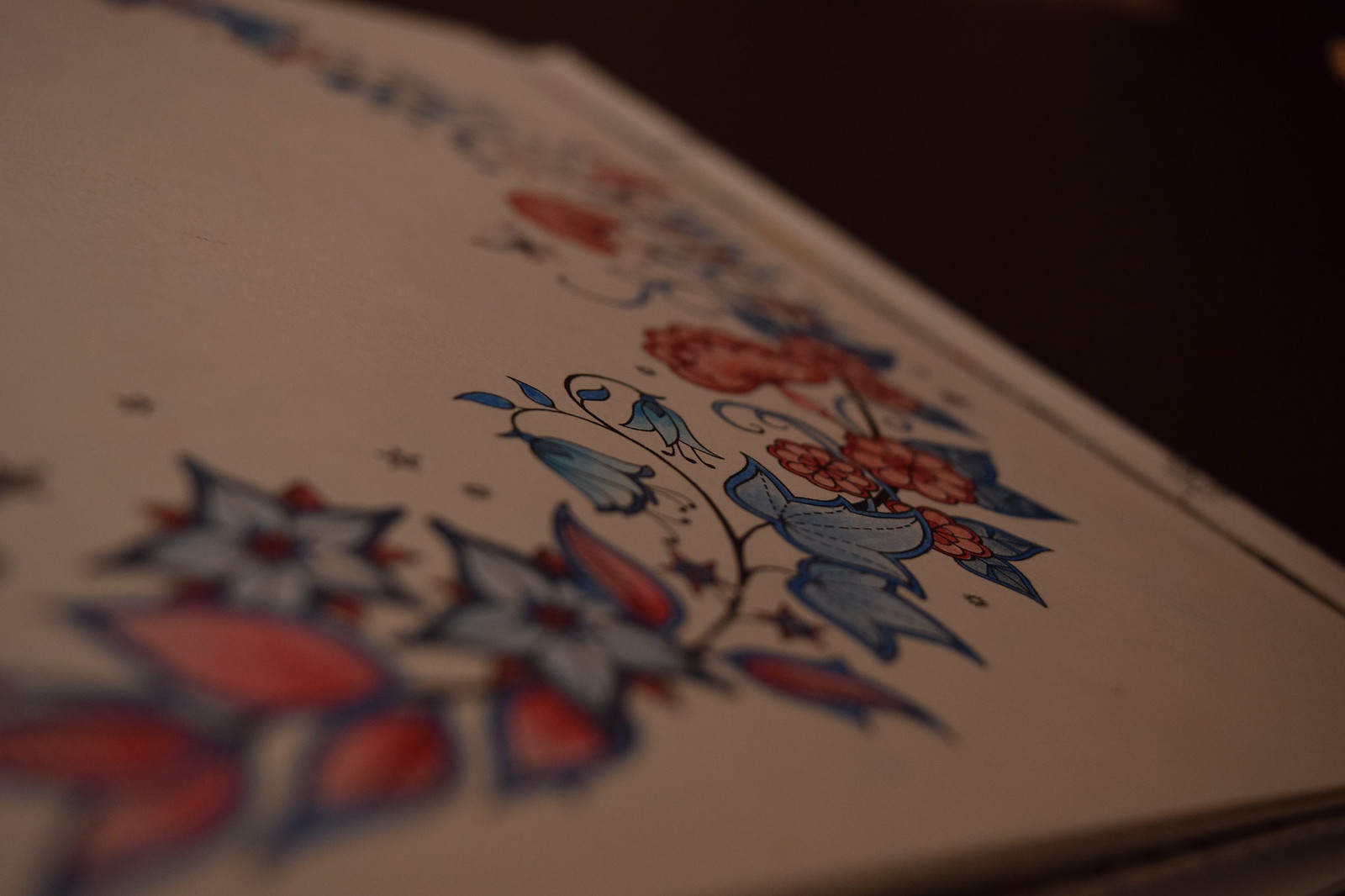The image depicts a close-up of a book cover, likely a notebook or scrapbook, set against an indistinct black background. The cover itself is predominantly an off-white hue, although it carries a reddish tint in the image. The design adorning the cover is intricate and features a vividly colored pattern that combines multicolored flowers and leaves. The floral design runs diagonally across the cover, with elements of foliage transitioning from dark blue to light blue hues, alongside vibrant red and orange flowers. The blue leaves are accentuated by a silhouette that darkens towards the edges, and the floral arrangement has an almost vine-like quality. A black line traverses the bottom of the cover, adding a final touch to the composition. The image suggests a thin book, possibly a child's book or a piece of artistic work, characterized by its detailed and carefully crafted botanical motifs.